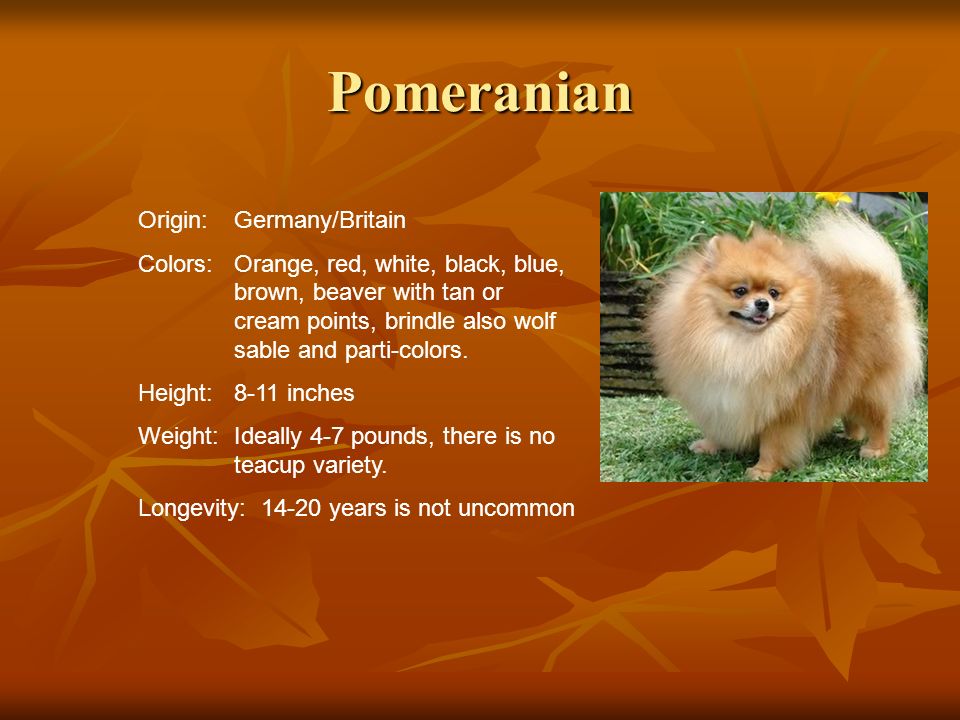This detailed image showcases a super fluffy Pomeranian dog with predominantly orange fur tinted with streaks of white. Positioned on a backdrop of grass, the Pomeranian sits against a vibrant, autumn-inspired orange background adorned with subtle yellow-orange leaves, contributing to a fall-like ambiance. Above the dog, the word "Pomeranian" is centrally placed at the top. The left side of the image is filled with descriptive text written in clear, white letters, detailing that Pomeranians originate from Germany and Britain and can come in various colors including orange, red, white, black, blue, brown, beaver with tan or cream points, brindle, wolf sable, and parti-colors. The text also provides information about their height (8-11 inches), weight (ideally 4-7 pounds), and longevity (14-20 years, with no teacup variety). Surrounding the dog are a few leaves, a yellow flower, and an object resembling a stone or wood, reinforcing the natural setting of the image. The overall presentation suggests the content might be from an informational book or a dedicated slideshow about Pomeranian dogs.